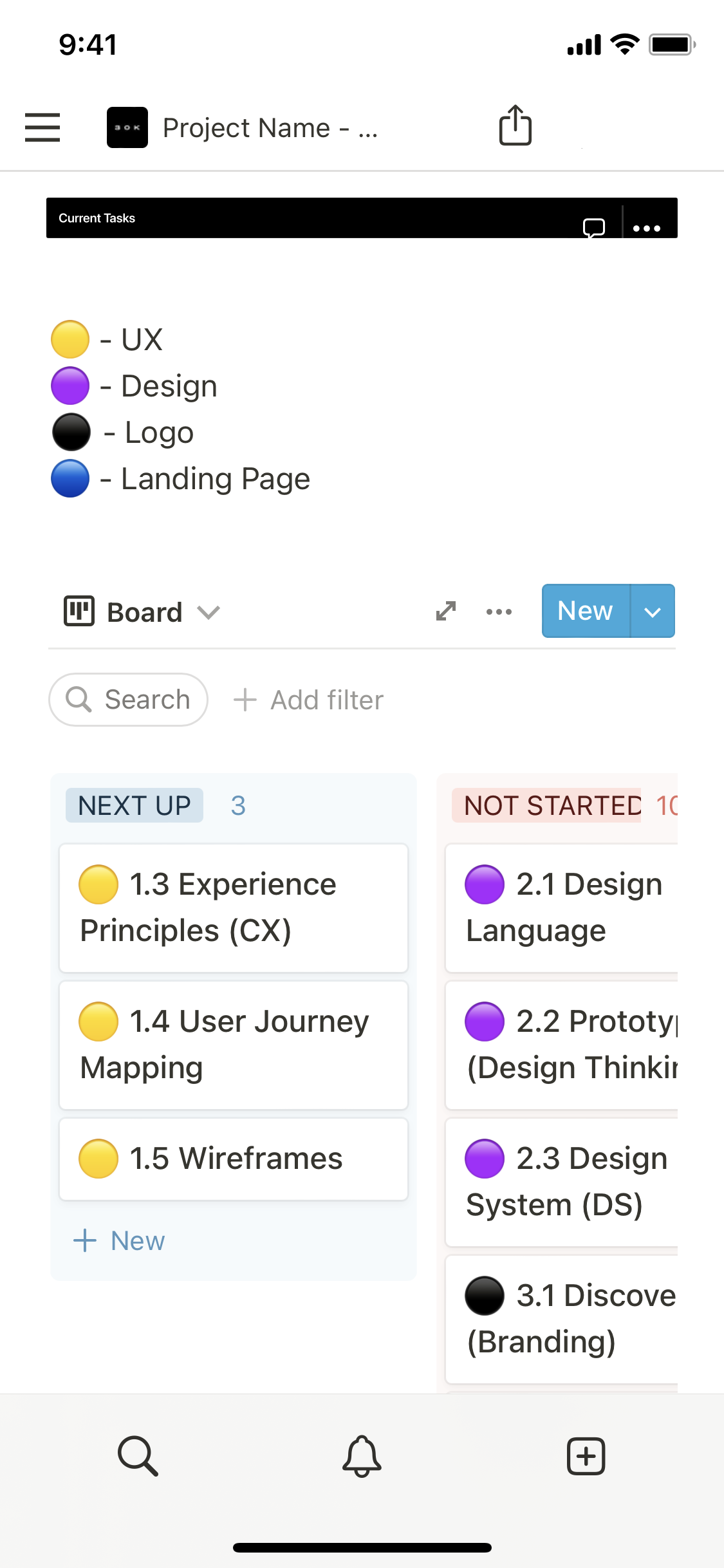This screenshot of a mobile application showcases a structured interface with various elements organized meticulously. 

The top of the screenshot features a white header adorned with black icons situated in the top left and right corners. On the left, there is a black hamburger menu, followed by a black square with rounded corners housing three white dots centrally placed. Proceeding to the right, there is dark gray text indicating the project name, followed by an ellipsis ("Project Name…"). After a brief section of negative space, a black outlined square with rounded corners, missing a portion on the top right side, contains a black arrow pointing upwards.

Beneath the header lies a thin light gray line, demarcating it from the main body of the page, which has a white background. Encapsulated at the top of the body section is a partially spanning black rectangle. On the left side of this rectangle, small white text reads "Current Tasks." On the right, three elements are arranged sequentially: a white outline of a speech bubble, a vertical white separator line, and three horizontally aligned white dots.

Following this rectangle is an area of negative space leading to a column of four colored orbs on the left side. Each orb exudes a gentle white shine at the top, transitioning to a solid color at the bottom. They are labeled in black text with corresponding colored orbs as follows: a yellow orb labeled “UX,” a purple one labeled “Design,” a black one labeled “Logo,” and a blue one labeled “Landing Page.” 

Further down, after another span of negative space, there's a black bar chart icon on the bottom left, indicating diverse bar heights protruding from the top. Adjacent to it, the word "Board" appears in black text, followed by a medium gray downward-pointing arrow. Situated in the bottom right corner of the page, dark gray arrows form an intersecting pattern, one diagonally pointing up and to the right, the other down and to the left at 45-degree angles.